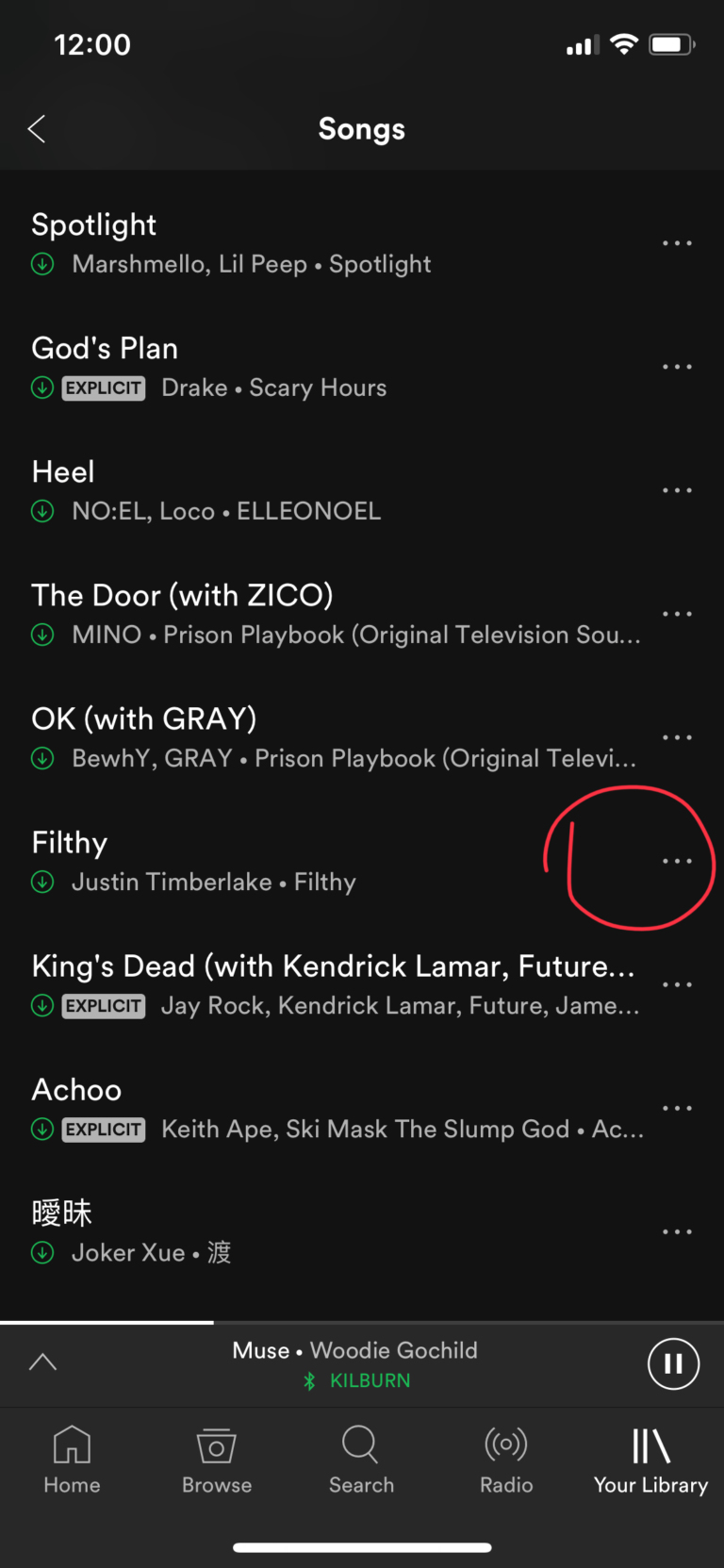The screenshot captures a section of the Spotify interface where the user appears to be browsing through a playlist or a set of saved songs. At the top of the list, notable tracks include "Spotlight" by Marshmello and Lil Peep, followed by "God's Plan" by Drake. Other songs featured are "Heal" by Noelle and Loco, "The Door" featuring Sicko by Mino, "Okay" with Gray by B.Y. Gray, "Filthy" by Justin Timberlake, "Kingston" featuring J-Rock, Kendrick Lamar, and Future, "Achoo" by Keith Ape and Ski Mask the Slump God, and a song in Chinese by Joker Xue. Notably, there is a circular highlight around the three vertical dots, or options menu, located on the right side of the song "Filthy" by Justin Timberlake, suggesting that the user might be intending to interact with this specific option.